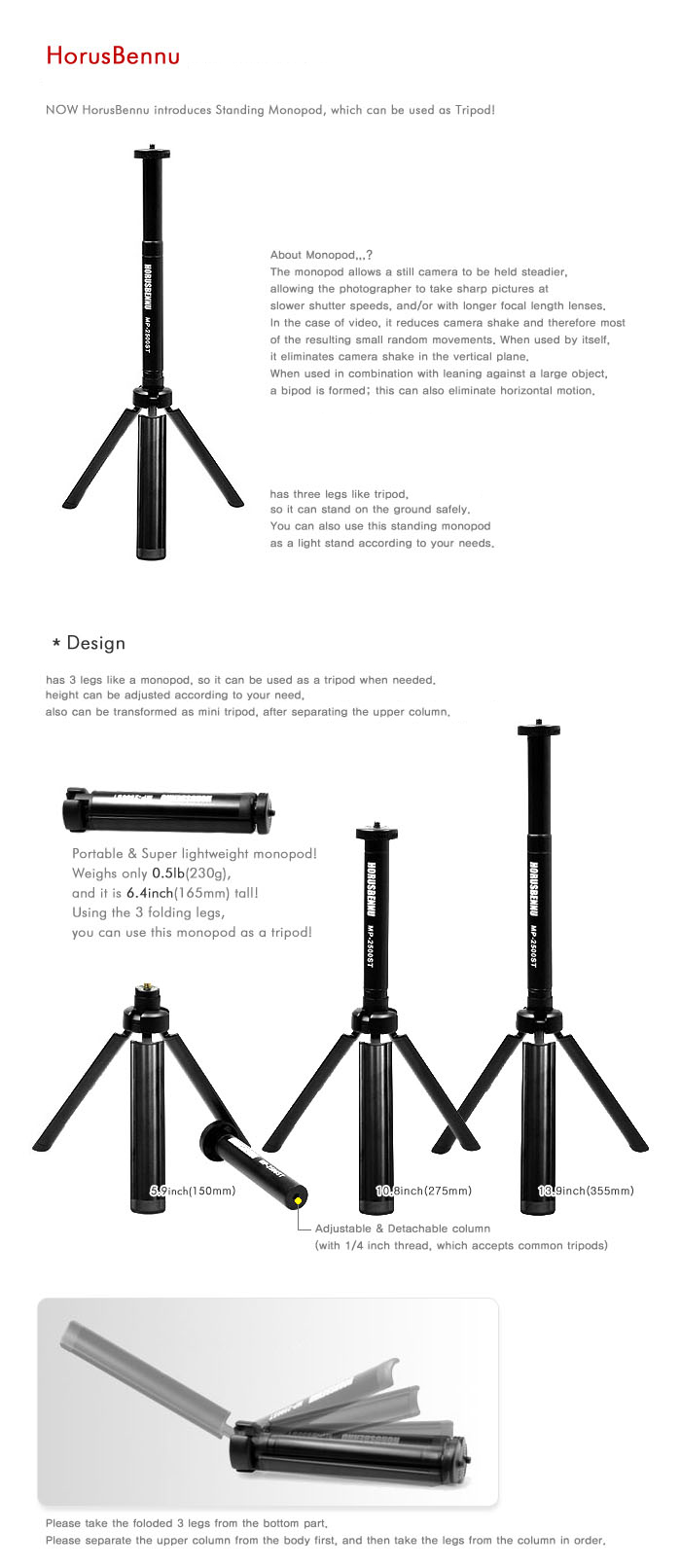The product image is a detailed promotional diagram for a Horace Bennu monopod, which can also function as a tripod. At the top, in red text, it reads "Horace Bennu." Below that, the introductory text in black states, "Now Horace Bennu introduces standing monopod which can be used on tripod." 

On the left side, a black monopod is prominently displayed, accompanied by two small paragraphs of descriptive black text. To the right of the monopod image, there is more descriptive text, although some of it is too small to read clearly. Below these sections, the word "design" is highlighted, followed by a description, likely detailing the monopod's weight and dimensions, although the exact wording is illegible.

The lower part of the diagram showcases the monopod in various states: one image illustrates the monopod completely folded up, while three additional images demonstrate the monopod extended to different heights. It's not clear whether this indicates a single adjustable product or three separate products of varying sizes. The entire layout rests on a white background, with the exception of one section that has a gray background. Despite the text's varying legibility, the visual representation effectively conveys the monopod's versatility and design features. The monopod itself is black, with some white text inscribed on it.